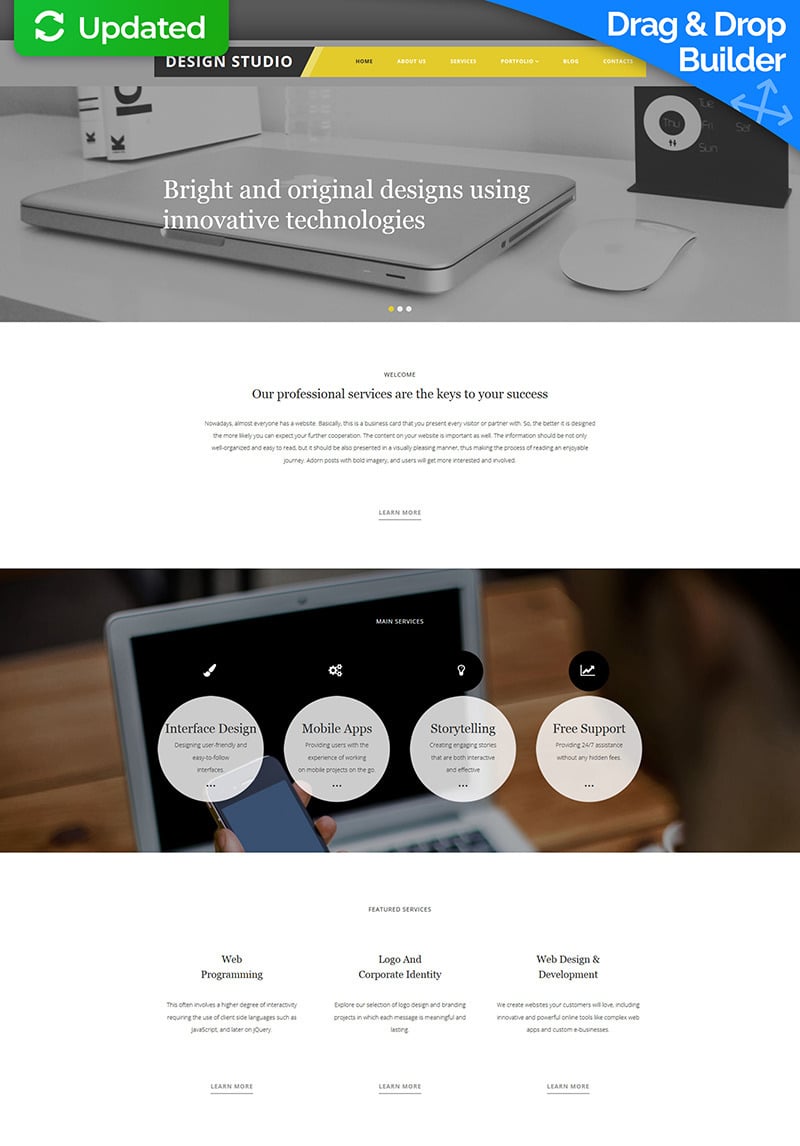Sure, here is a clean and detailed caption for the given image:

---

The screenshot displays a user interface for a design tool. The top banner is blue and features the text "Drag and Drop Builder" accompanied by a multidirectional cross-arrow icon. In the center of the image, there is a pop-up notification framed in a mock-up style, stating, "Updated," with the text written in italics. Below the pop-up, the title "Design Studios" is prominently featured in black text. A yellow search bar is visible beneath the title. A paragraph of text explains the tool's purpose: "Write an original design using innovative technology and professional services are the key to your success." Below this section, images of a phone and a computer are shown, with accompanying text that reads: "Interface Design, Mobile and Web Programming, Local and Corporate Identity, Web Design, and Development."

---

This detailed and cleaned-up caption captures all the essential elements described in the voice input.